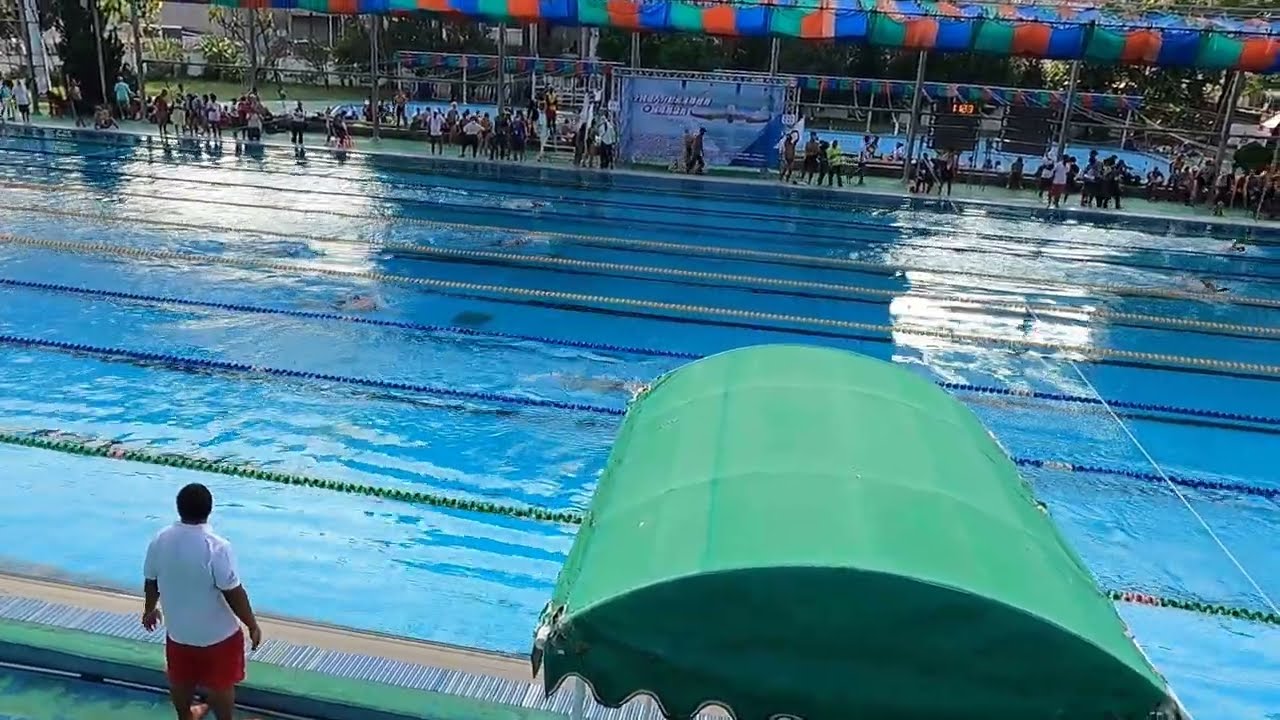The image depicts an overhead view of a high-level swimming event set in an outdoor pool, featuring multiple lanes, possibly 9 or 10, designed for competitive racing. In the bottom left corner, a man, likely the lifeguard, is standing at the pool’s edge. A large green canopy or overhang is prominently featured in the bottom portion of the image, providing partial cover to the pool area. The pool occupies the center of the image, stretching from left to right, and appears overall empty. Towards the top, various spectators and competitors can be seen milling about, without formal seating arrangements, just lounging by the pool. The setting is accentuated by the presence of various colors including white, red, light blue, green, dark blue, and gray. In the distance, there are some ribbons, fences, and indistinct text from posters, suggesting the presence of event signage. The scene is clearly captured in the middle of the day.